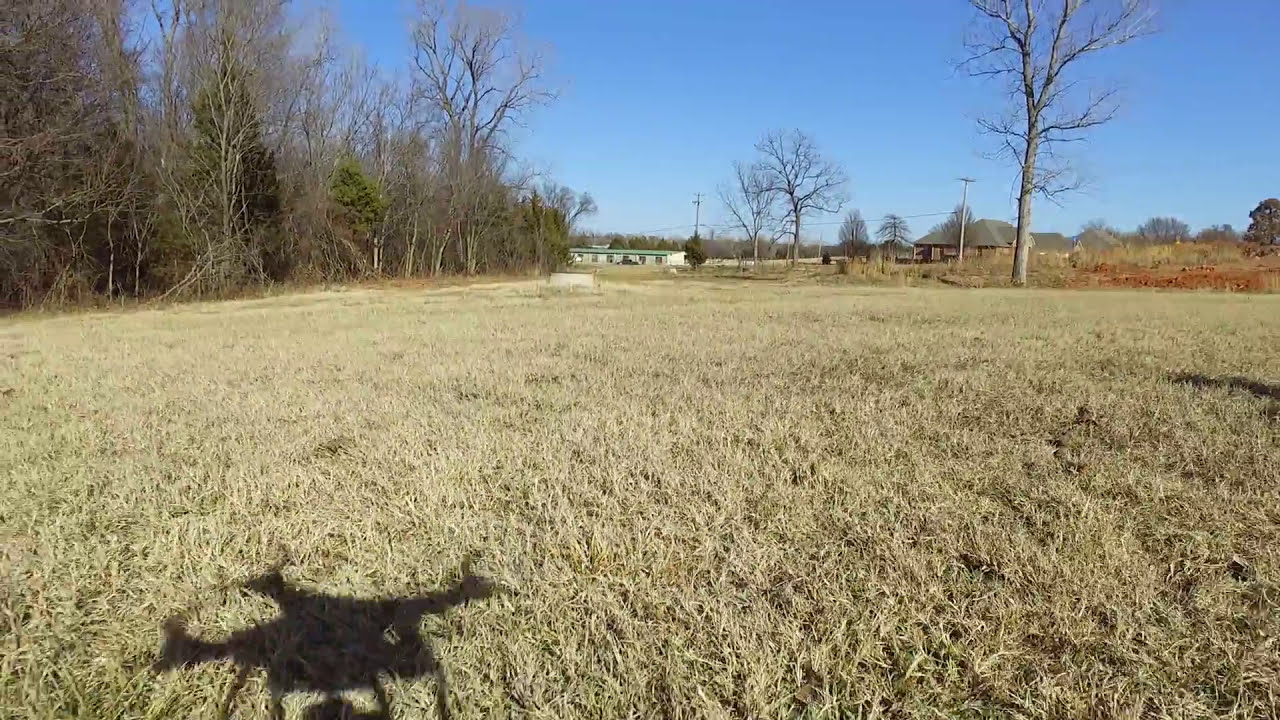This aerial image, captured by a drone as indicated by its shadow in the bottom left corner, depicts a sprawling, dry grassy field that suggests a fall or winter setting. The grass is brittle and brown, giving the landscape a desolate, cream-colored appearance. To the left, there is a sparse forested area with mostly barren trees, though a few evergreens and some trees with lingering green leaves are visible. On the right side, the landscape transitions into agricultural land with low-lying brown grasses and a few leafless straggling trees. In the background, some houses and structures can be seen, providing a sense of human presence. The sky above is a clear, uninterrupted blue, contrasting with the earthy tones below.